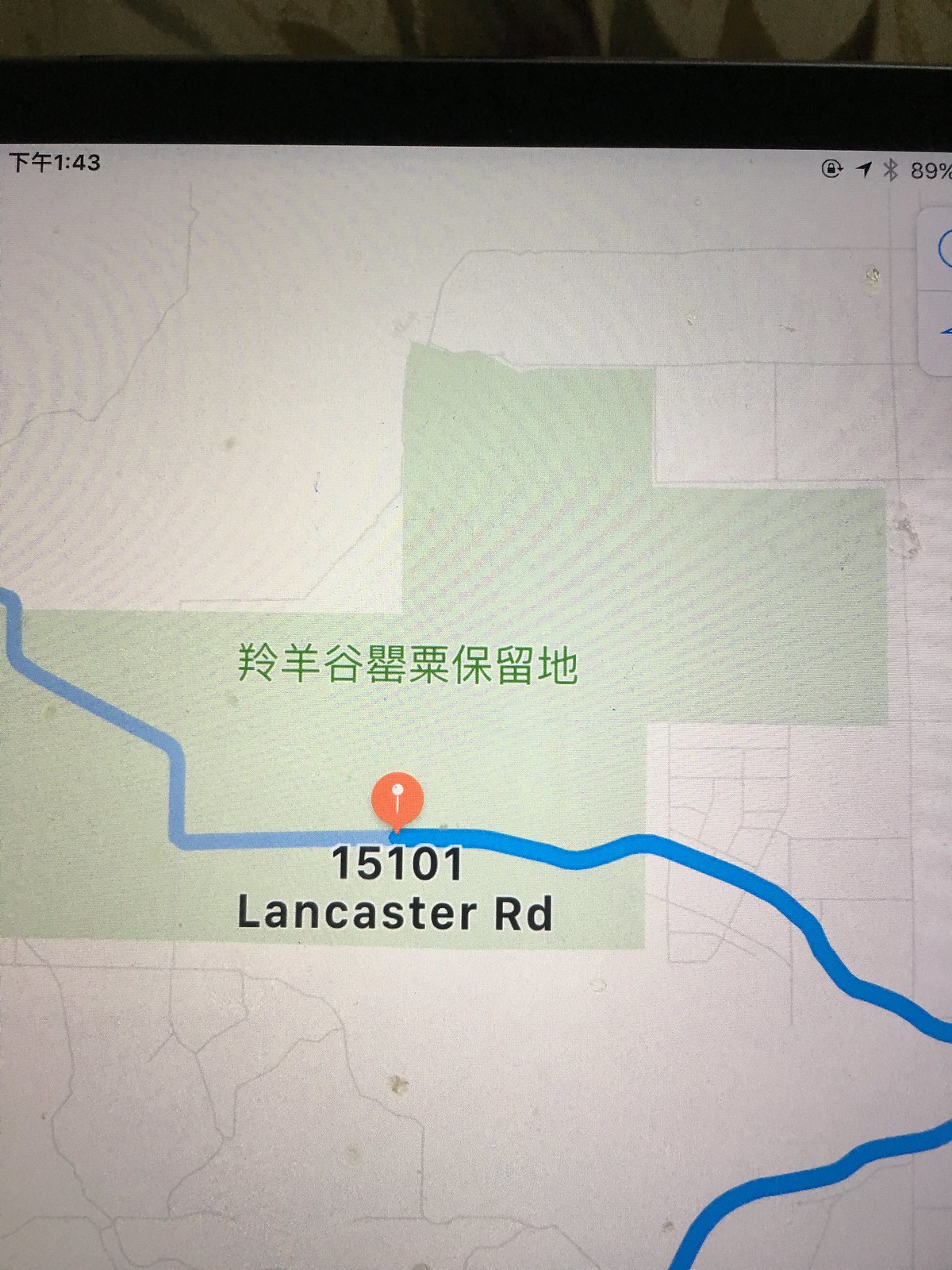The image is a detailed color photograph of a tablet or cell phone screen displaying a close-up of a Google Maps page. The map features a predominantly white background with numerous gray lines representing streets. In the center of the screen, there's a notable green, blocky section resembling a dog in shape, with Asian writing, possibly kanji or Chinese, in the middle of the green area. A prominent red pin marks the destination labeled as "15101 Lancaster Road." A blue navigation path starts from the left edge of the screen, curves downwards, and extends to the bottom of the image, indicating the route to the destination. At the top of the screen, the time reads "1:43," and the battery charge is indicated at 89% along with a Bluetooth icon. The image also captures part of the surrounding environment, with a hint of a pillow visible in the background.